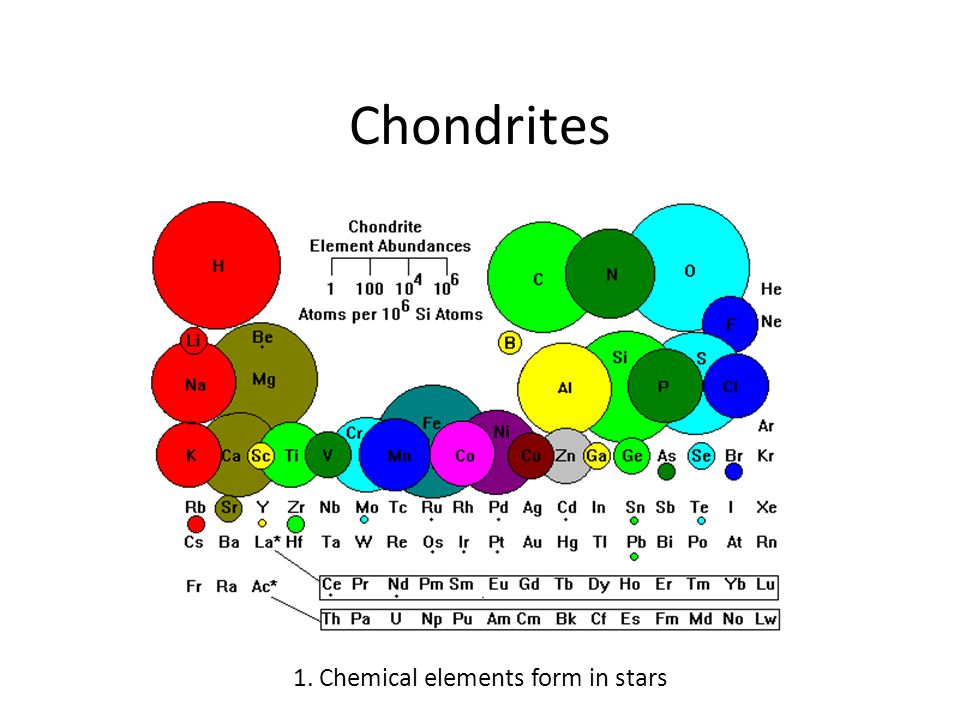The image is a detailed scientific infographic resembling an elemental chart, titled 'Chondrites' in black text at the top. The chart, set against a white background, features abbreviated chemical elements, some labeled with sequences such as 'm-b-m-o-t-c-r-u-r-h-i-r-o-s-r-e-w-t-a.' A distinctive color-coding system is used, with vibrant bubbles or circles ranging in size and hues, including shades of green (lime, leaf, olive), red, yellow, teal, blue (cerulean, dark, light, bright), purple, pink, gray, and dark burgundy. At the bottom of the chart, there's a notable designation: 'Number 1' followed by the sentence 'Chemical elements form in stars,' indicating the origin of these elements. Additionally, a quantitative scale marks the abundance of these chondrite elements, annotated as '1, 100, 10^4, 10^6 atoms per 10^6' to illustrate their distribution. The overall layout is organized yet scattered, providing an intricate visual representation of the chemical makeup akin to a refined periodic table.